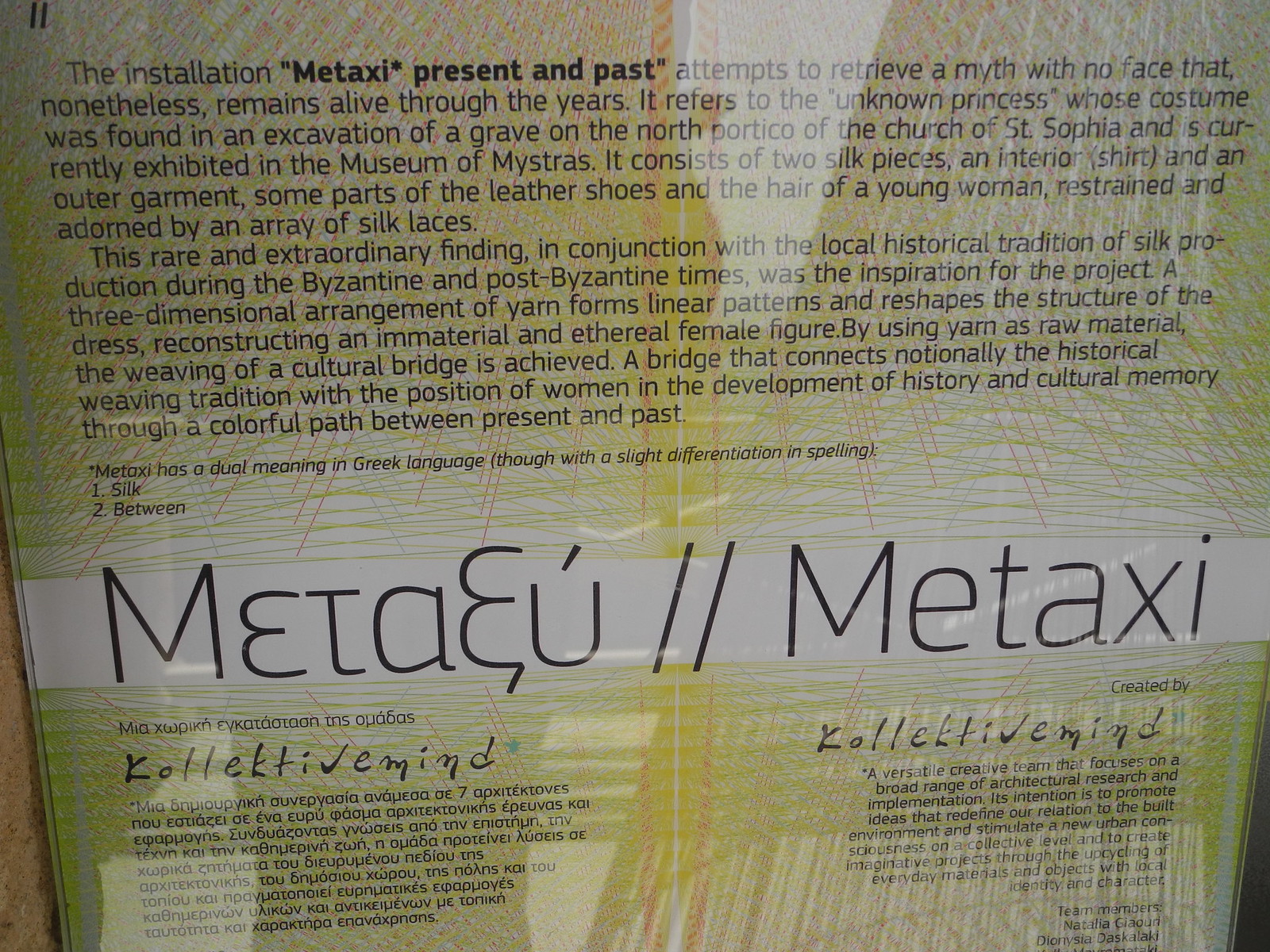The image depicts a detailed plaque, positioned behind glass, describing an art installation named "Metaxi." The photograph, taken outdoors in a historical site during the day, shows a close-up, front-facing view of the sign. The plaque is colorful, featuring shades of black, white, brown, green, yellow, and orange. 

The text on the plaque, presented in both English and Greek, explains the installation "Metaxi, Present and Past." It attempts to retrieve a myth with no face that remains alive through years. The installation refers to an unknown priestess, whose costume was found during an excavation at the north portico of the Church of St. Sophia and is now exhibited in the Museum of Mystras. It comprises two silk pieces: an interior shirt and an outer garment. Additional details include leather shoes and hair adorned with silk laces from a young woman, forming a rare archaeological find. 

This installation draws inspiration from local historical silk production during Byzantine and post-Byzantine times. A three-dimensional arrangement of yarn reconstructs the priestess's dress, weaving a cultural bridge that melds historical weaving traditions with the role of women in history. The word "Metaxi," with its dual meanings in Greek—“silk” and “in between”—symbolizes this connection across time.